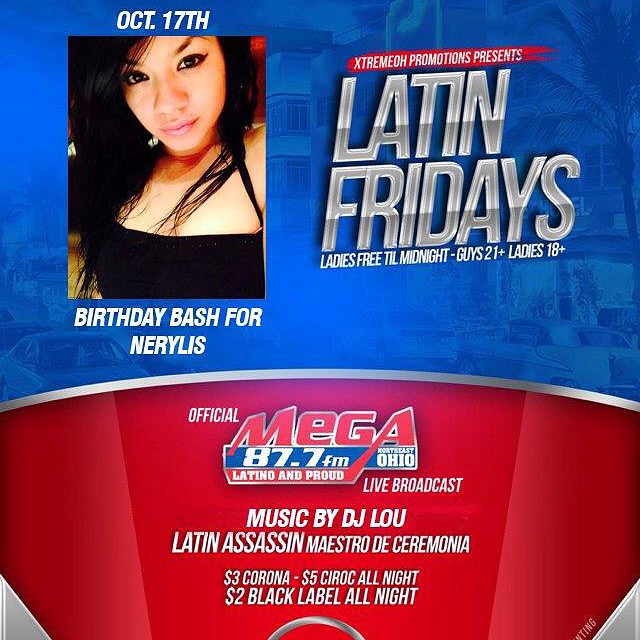The advertisement prominently features a festive promotional poster for a club party. The left side of the poster is primarily blue and showcases an attractive woman with dark hair, likely of Latin American descent, dressed in a black top. She gazes slightly downward. Above her image, it reads "October 17th," indicating the event date. Below her, there is a caption: "Birthday Bash for Nerilis."

On the right side, the poster, transitioning to red at the bottom, announces "Xtreme DH Promotions presents Latin Fridays." The details indicate that ladies gain free entry until midnight, while the age requirements are 21+ for men and 18+ for women. The lower section, bordered by a silver band in an arc, highlights "Official Mega 87.7 FM, Northeast Ohio, Latino and proud." It confirms a live broadcast featuring music by DJ Lou and Latin Assassin as the Maestro de Ceremonia. Additionally, promotional drink specials are listed: $3 Corona, $5 Ciroc, and $2 Black Label all night. The bottom design includes a silver ring resembling part of a dial, flanked by silver-colored triangles enhancing the festive aesthetic.